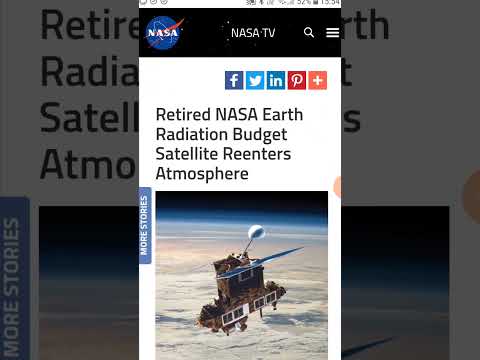The image comprises two sections. The background features a close-up of a webpage showing a slightly visible news article with a white background and large bold black text. The only legible word is "retire," along with a partial reference to "satellites." The webpage is mostly obscured but suggests an article about a satellite retirement.

In the foreground, there's a detailed screenshot. At the top, a white background displays several black icons including a Wi-Fi signal, battery status, and the current time. Below these icons, a black banner features a blue globe with "NASA" written in white, accompanied by a red mark that says "NASA TV." A magnifying glass icon with white lines is also present. Moving down, a series of social media icons appear in blue and white for Facebook, Twitter, and LinkedIn, a red and white Pinterest icon, and a salmon-orange box with a white plus sign.

The main headline reads: "Retired NASA Earth Radiation Budget Satellite Reenters Atmosphere." Below the headline is an image of a satellite. The satellite is brown, shaped somewhat like a house with white window-like structures, and features a protruding solar panel. A bulky white structure that looks like an antenna is mounted on top. The satellite appears to be floating over Earth, which is depicted with visible cloud cover, brown landmasses, and a black and blue horizon. To the side of the image, a blue banner reads "More Stories."